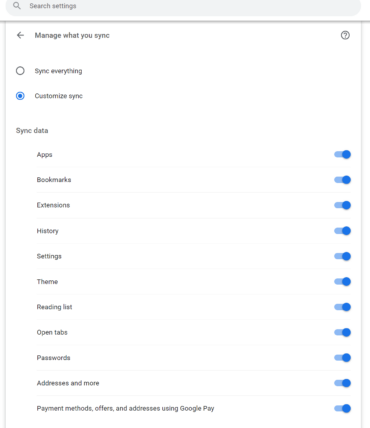In the image, a settings interface of a tablet or phone is displayed. At the top center, there is a search bar featuring a magnifying glass icon on the left and the text "Search settings" in light gray color on the right. Directly below, the phrase "Manage what you sync" is shown, flanked by a left-pointing arrow on the left and a circle with a question mark on the far right.

Moving downwards on the left side, two synchronization options are presented. The first option, "Sync everything," is accompanied by an empty circle on its left. Below this, the option "Customize sync" appears, marked by a blue-filled circle to its left.

Further down on the left side, a dedicated "Sync data" section lists multiple categories for synchronization. These categories include "Apps," "Bookmarks," "Extensions," "History," "Settings," "Themes," "Reading List," "Open Tabs," "Passwords," "Addresses and more," "Payment methods," "Offers," and "Addresses using Google Play." Each category is paired with a small check box located to its right.